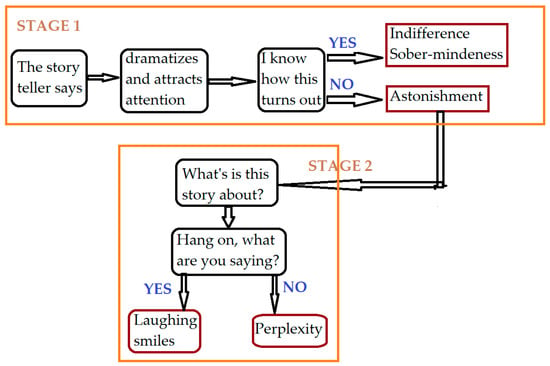The image is a detailed flowchart on a white background, likely found in a notebook or textbook, illustrating the process of storytelling in two stages. The flowchart is split into Stage One and Stage Two.

**Stage One** is depicted in a long orange-bordered rectangle at the top. It begins with "The storyteller says" in the first box, followed by an arrow leading to the next box that states "Dramatizes and attracts attention." Another arrow points to "I know how this turns out," which branches into two options: "Yes," leading to "Indifference, sober-mindedness," and "No," leading to "Astonishment." An arrow from "Astonishment" directs downwards to Stage Two.

**Stage Two** consists of a box labeled "What's this story about?" with an arrow pointing down to "Hang on, what are you saying?". This then branches into "Yes," leading to "Laughing smiles," and "No," leading to "Perplexity."

Overall, the flowchart visually represents the steps and decision points in creating and understanding a story, highlighting the storyteller's role in engaging the audience and the audience's possible reactions.